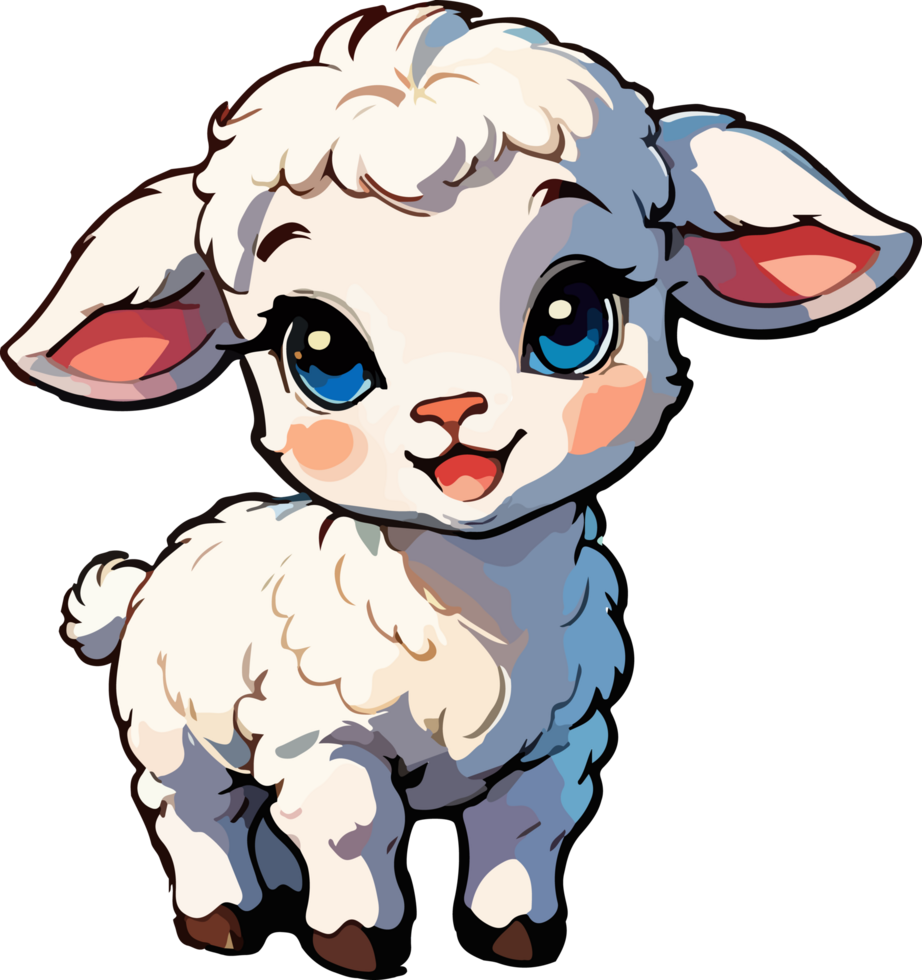This image features a cartoon-style depiction of a baby lamb viewed from the front. The lamb has a very expressive face with large, bright blue eyes adorned with black eyelashes, and rosy, peach-colored cheeks. Its mouth is open, revealing a pinkish-red tongue, and it has a small orange nose. The lamb's ears are large and fluffy, starting off white and transitioning through shades of dark and light purple to a salmon-colored pink on the sides.

The lamb’s body is covered in light, fluffy fur, with a white mop of hair on its head. Its torso, which tints light blue on the right side, has a soft light pinkish-white color overall. The lamb’s underbelly is shaded dark gray, giving the impression of a shadow. It stands on chunky legs with brown hooves, and its bushy tail is white with a hint of dark gray at the tip. The entire lamb is outlined in a black line, enhancing the sketch's details. The setting is simple with a plain white background, giving all the focus to the adorable animated character that might belong to a children’s nursery rhyme or story.